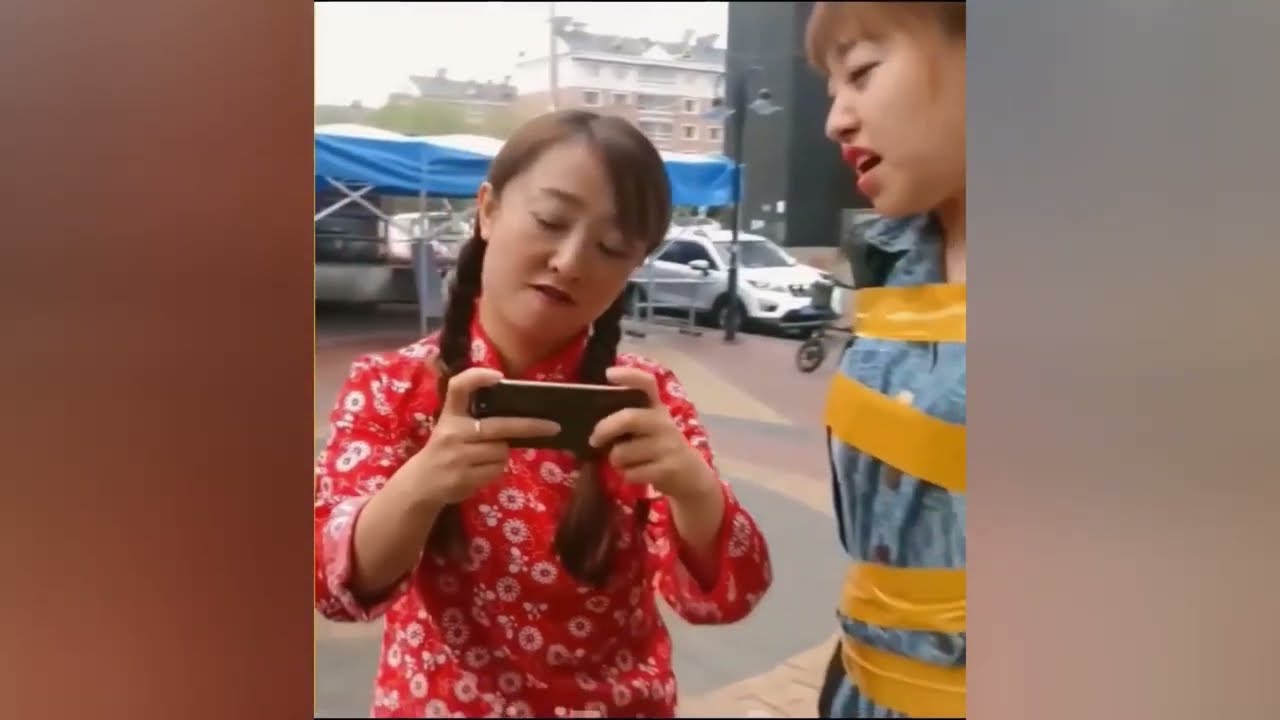The image depicts two Asian women standing outside on a street during the daytime. The picture is horizontally rectangular with vertical solid-colored borders: brown on the left and gray on the right. The woman on the left has long, brown, braided hair with bangs and is wearing a red top adorned with a white floral pattern, her sleeves rolled up to her elbows. She holds an iPhone horizontally in both of her hands, intently looking down at it. To her right stands a taller woman with short brown hair and bangs, her mouth agape as if in distress. She is dressed in a blue button-down shirt and appears to be wrapped in wide strips of yellow tape. The background features a slightly blurred white car parked beside a street, a blue tent with a matching awning, a distant building, and trees under a clear sky. The overall scene is brightly illuminated by natural light.